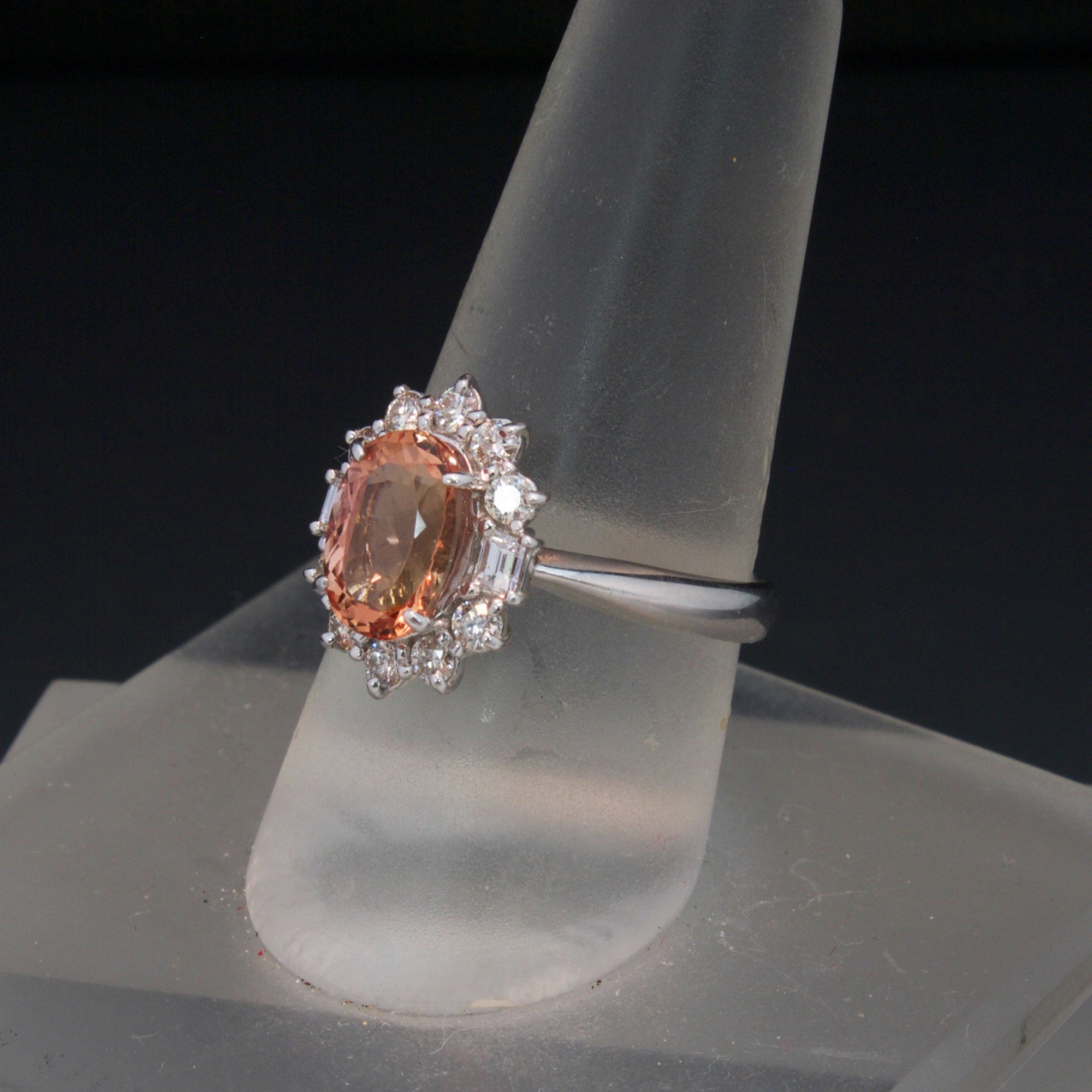Against a featureless black backdrop, a silver ring is displayed prominently on a scratched and dirty gray plastic stand, resembling a tapered plexiglass rod that ascends slightly to the right before extending off the top of the image. The ring's band is silver, featuring a central egg-shaped orange ruby held by four prongs. Surrounding the ruby, the outer part of the band boasts an intricate floral motif, with each tiny flower embedded with a diamond at its center. The overall setup creates a striking contrast between the gleaming details of the ring and the hazy, sanded appearance of the stand.